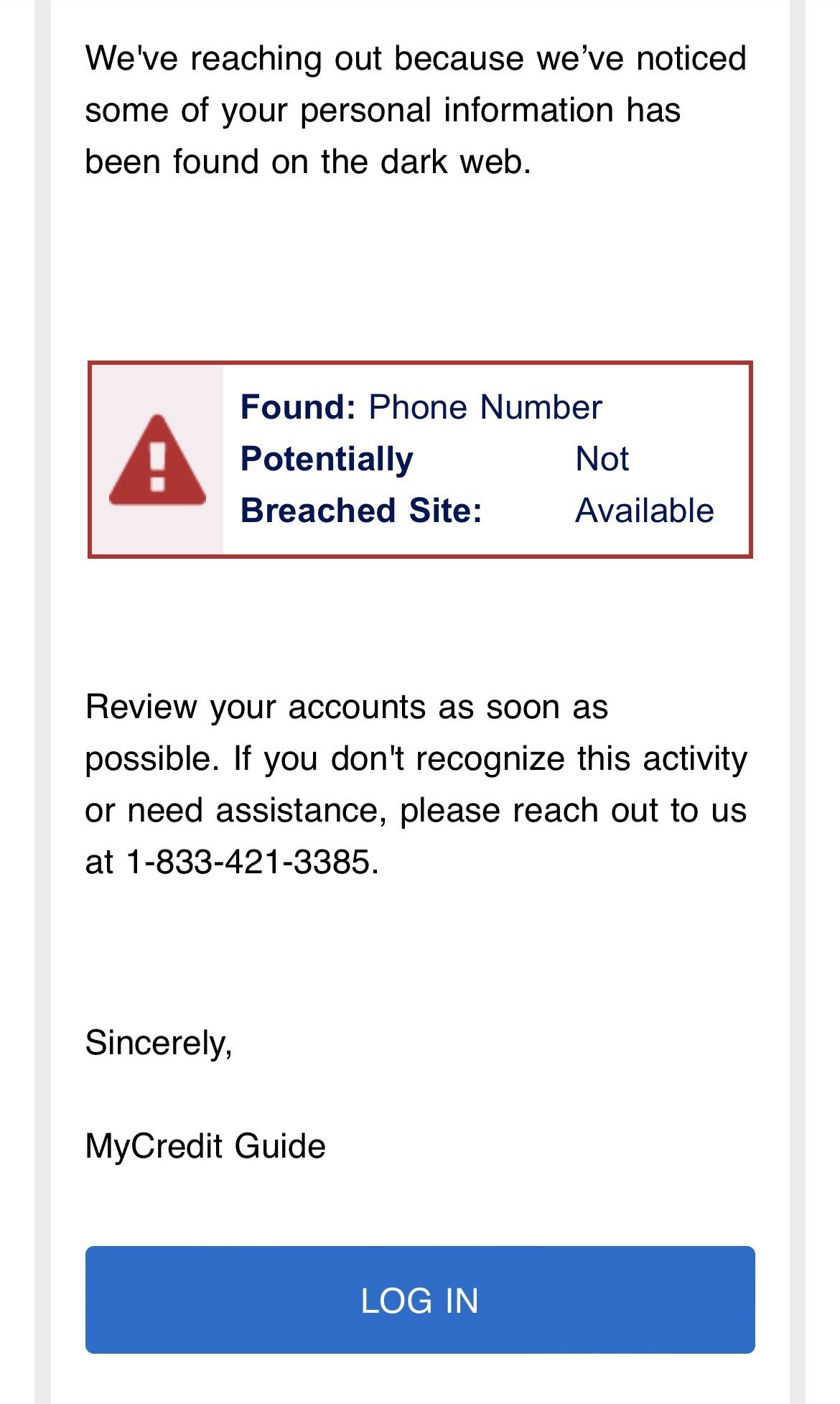This is a detailed caption for the given image:

---

This image is a screenshot from a mobile application, displaying a notification message on a white background with black text. The primary message informs the user that some of their personal information has been found on the dark web. Below the main message is a red box containing a disclaimer, outlined in red, with text stating: "Found: a phone number. Potentially not breached site available." Beneath the red disclaimer box, additional text advises the user to review their account immediately if they do not recognize the activity or need assistance. It provides a contact number: "1-833-421-3385" and concludes with "Sincerely, My Credit Guide" (formatted as two separate words). At the bottom of the screenshot, there is a blue login button for user interaction. The overall layout includes three sections, but these sections are distinguished by spaces rather than explicit divisions. 

---

This caption offers a thorough description of the visual components and textual information present in the screenshot.